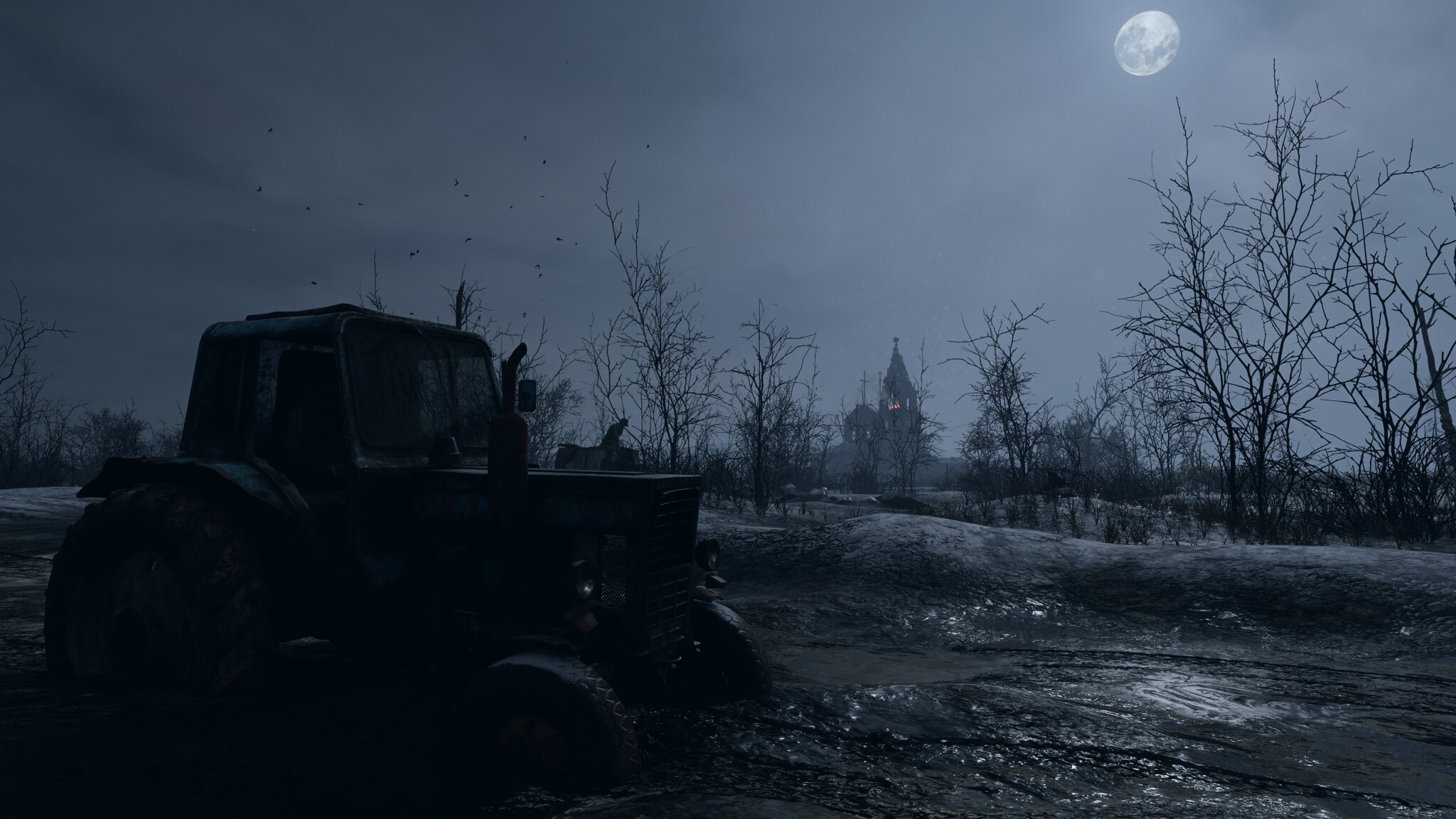A surreal and eerie night scene captures an off-road vehicle trapped in thick, brown mud in the foreground, its large black tires partially submerged. Overhead, the softly glowing moon peeks through a partially cloudy sky, casting a serene light on the slick mud. A subtle reflection of the moonlight shimmers in the mud puddle below. In the sky, a small flock of birds adds a haunting element to the image. Bare, skeletal tree branches stretch ominously in the middle ground, adding to the desolate atmosphere. Looming in the distant background, a mysterious castle stands out, illuminated by an eerie orange glow from its windows, enhancing the night’s mystique. The combination of natural elements and the unexpected castle backdrop creates a chilling, otherworldly scene.